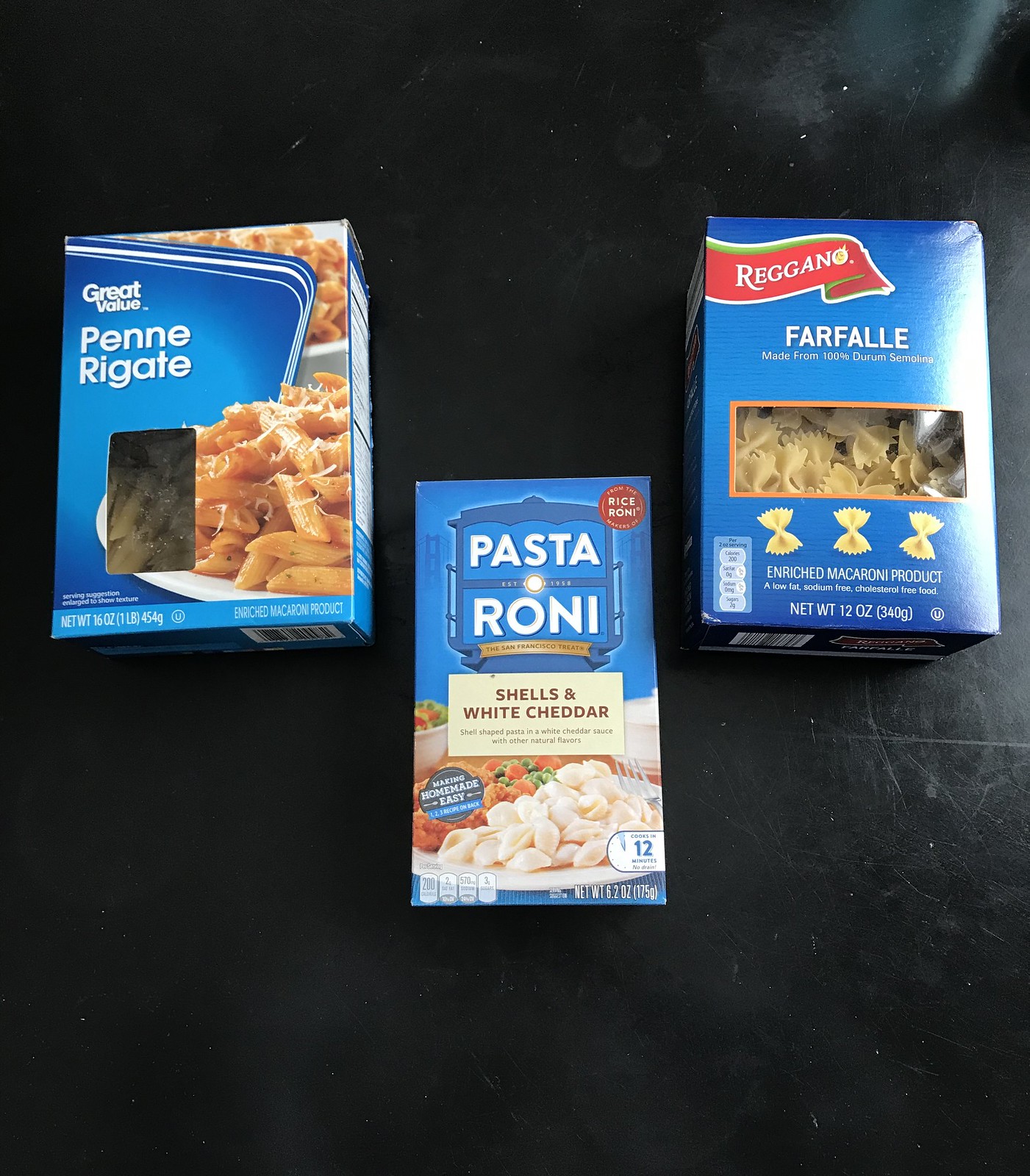In the image, three boxes of pasta are displayed on a black countertop with faint grayish stains. Each box is blue but from distinct brands, suggesting a potential comparison photo. 

The first box on the left is labeled "Penne Rigate" from the brand Great Value. The box displays an appetizing pile of yellow penne noodles on a plate. 

The middle box is from Pasta Roni, featuring "Shells & White Cheddar." A picture on the box shows white pasta shells smothered in creamy white cheddar, accompanied by other food items.

The far-right box is labeled "Farfalle" from the brand Reggiana, prominently featuring a red banner. Through a window on the box, bowtie-shaped pasta is visible. Additional images of three yellow bowtie pastas are depicted on the box itself.